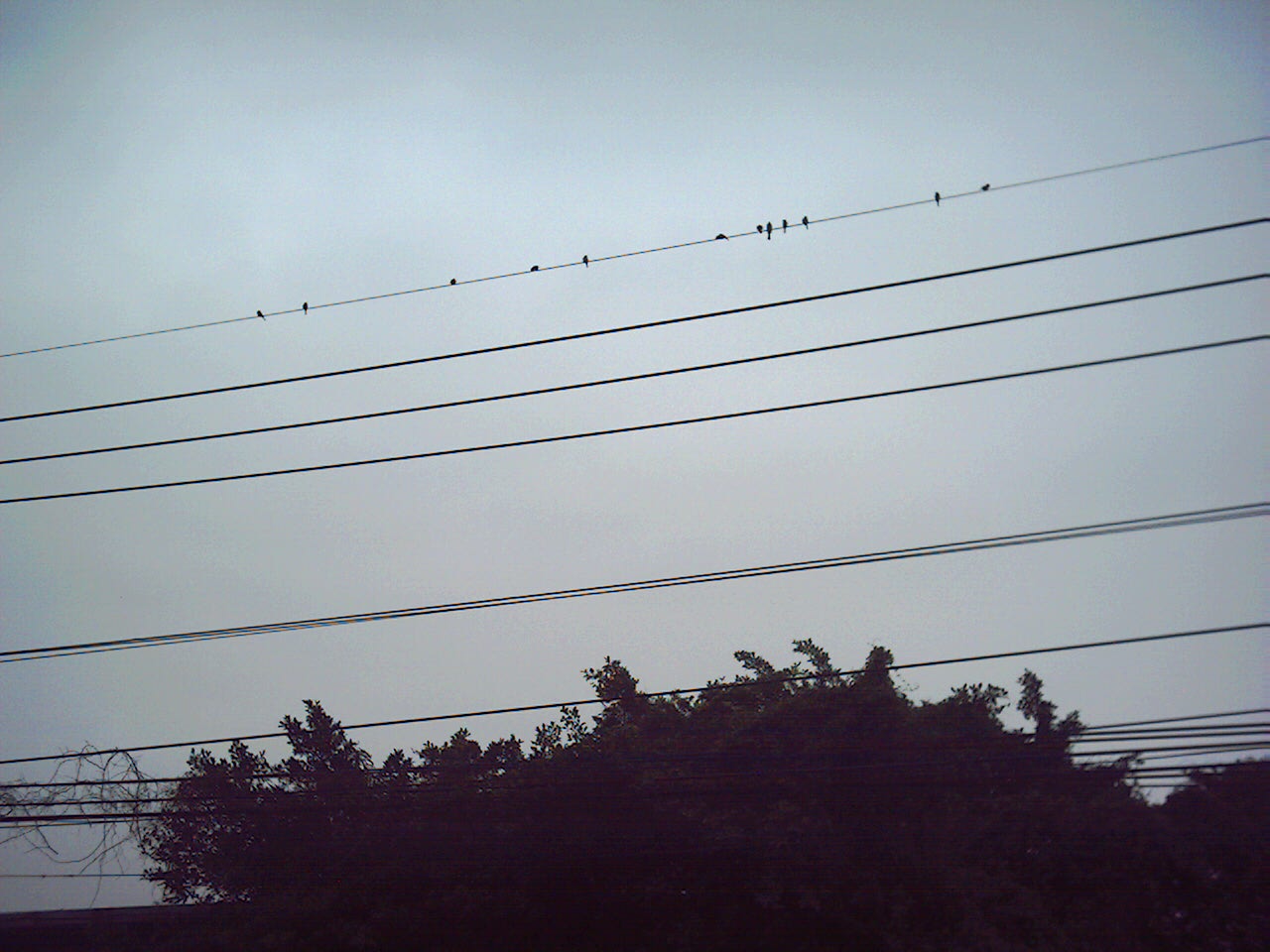This color photograph, taken outdoors during a possibly overcast day with a misty gray sky, presents a tranquil yet somber scene. The sky is uniform in its overcast appearance, devoid of distinct cloud formations, casting a subdued light across the landscape. At the bottom of the horizontal rectangular frame, the dark silhouettes of tall trees form a shadowy boundary, their details obscured in the dim light. Spanning the width of the image are numerous telephone lines, creating a linear pattern across the scene. The topmost line is particularly thin and hosts a flock of small birds – precisely twelve in silhouette. Below, several thicker lines are grouped closely together, adding to the structured complexity of the composition. The photograph lacks any additional elements such as text, people, buildings, vehicles, or other animals, offering a pure, undisturbed glimpse of this serene, minimalist landscape.